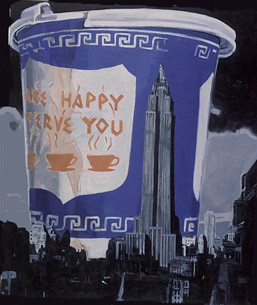The image depicts a rectangular painting dominated by a cityscape with dark color palettes of blacks and grays. The foreground features a tall, pointy skyscraper that serves as the focal point, almost reaching the top of the canvas. Below the skyline, there is a street lined with trees and a visible white line running through it.

In the background, a colossal blue coffee cup, reminiscent of Greek-themed designs, dwarfs the city. This cup features intricate white embellishments, including wave-like lines and a decorative geometric border at the top and bottom. The cup also showcases a white shield with the phrase "We Are Happy to Serve You" in orange lettering, partially obscured in some areas. Additionally, the shield displays three orange coffee cups emitting steam.

The scene behind the cup transitions from a black upper section to a lighter gray and white area, suggesting a cloudy sky. These visual elements create a contrast between the dark urban foreground and the lighter, more whimsical background dominated by the oversized, ornate coffee cup.